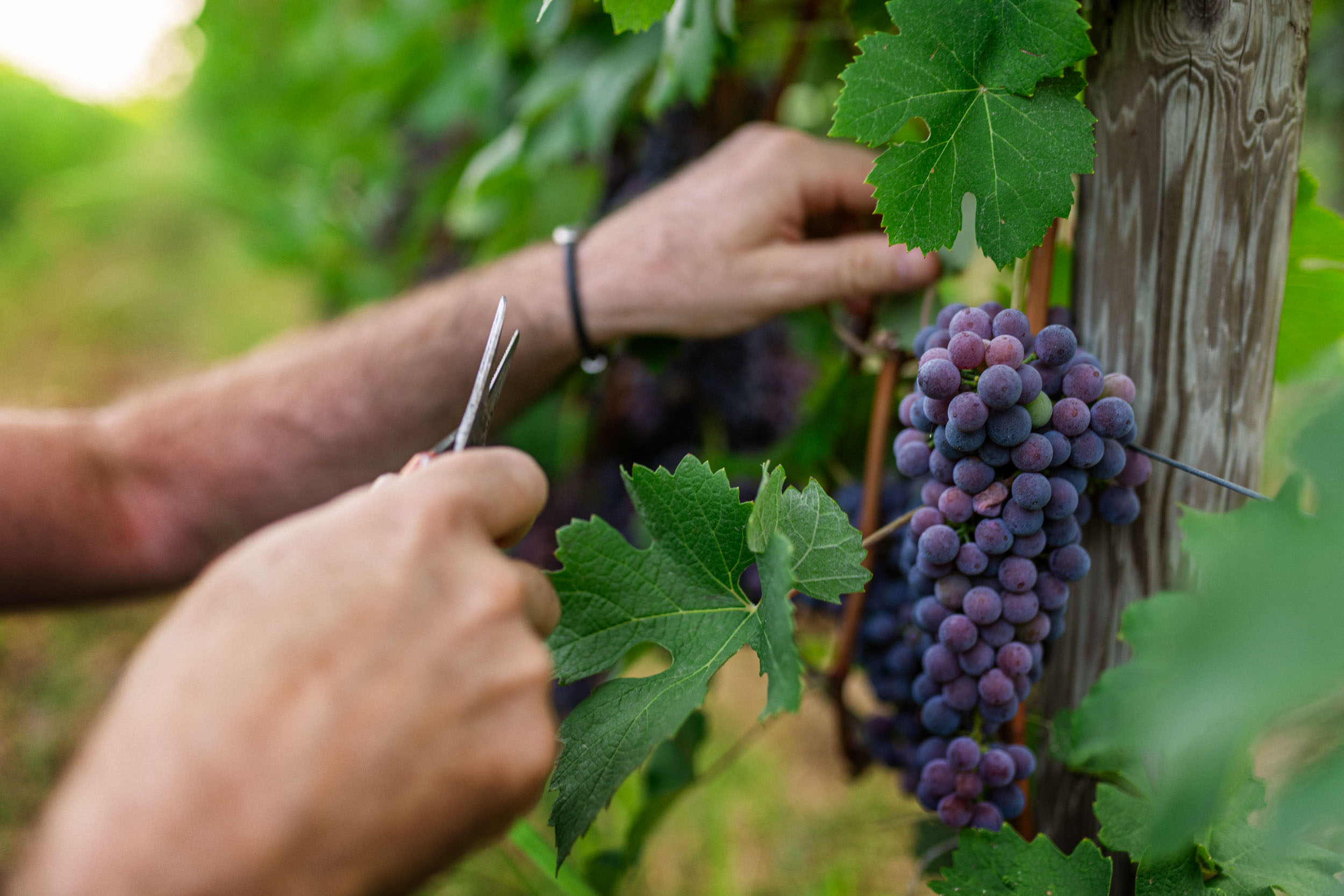In this vivid outdoor image, a man is meticulously harvesting grapes in a lush vineyard. The extreme background is blurred, rendered in multiple shades of green, providing a serene ambiance to the scene. The focal point of the image is the vibrant grapevine adorned with green leaves and a lone, enticing cluster of ripe purple grapes. On the left side of the image, the man's unsleeved left arm, noticeable by its hairiness, wears a minimalist rawhide tie bracelet accented with two lighter-colored beads. His right hand, intent and precise, grasps a silver pair of scissors, poised to cut the grapes from the vine. His left hand steadies the stem, ensuring a careful and clean cut. The grapes themselves are a striking mix of purples and blues, indicating their ripeness and freshness. In the blurred background, the vineyard stretches into rows, suggesting the vastness of the grape-growing area and the dedication to cultivating these fruits, possibly for wine production or fresh market sale. The image captures the meticulous care and tranquil beauty of grape harvesting in this sunlit vineyard.